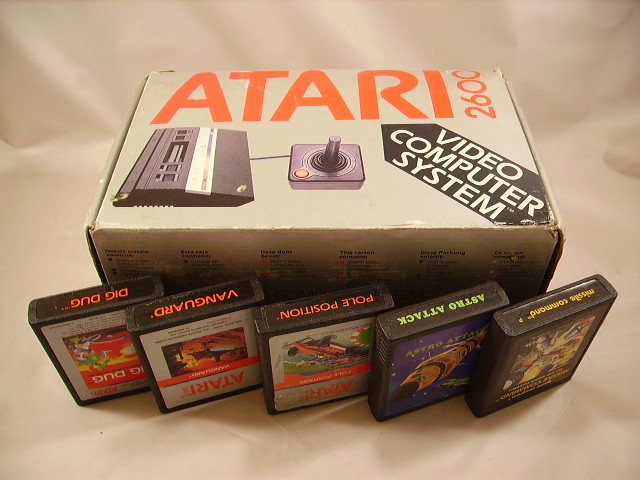The photograph captures an Atari 2600 Video Computer System in its original packaging, prominently featuring "Atari" in large orange text on the upper half and "2600" vertically below. Overlaying the corner is a banner reading "Video Computer System." The box’s illustration showcases the rectangular console and a joystick controller. The entire scene is set against a somewhat crumpled, beige-colored backdrop, likely paper or stiff grey cloth. In front of the box, five black game cartridges, roughly the size of a deck of cards, are neatly arranged. These cartridges are for the games Dig Dug, Vanguard, Pole Position, Astro Attack, and Missile Command. The photograph, taken indoors with a standard camera, offers a nostalgic glimpse into vintage gaming from the late 1970s to 1980s.